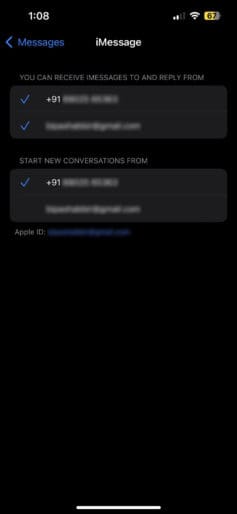This screenshot, captured from an Apple mobile device, showcases an interface display typical of the iMessage settings. Along the top of the screenshot, standard icons for smartphone usability are visible, including the time, network connection status, Wi-Fi signal, and battery life indicator. The background of the display is black, highlighting the focus on the iMessage settings information presented.

The screenshot specifically includes details on iMessage, featuring a section navigated from the main Messages menu. In it, the user can see options related to receiving messages and starting new conversations. Critical personal information, such as phone numbers and email addresses, has been deliberately blurred for privacy. These sections provide instructions and options for message reception, including the blurred phone number and email addresses, along with a prompt to start new conversations from the listed contact details.

At the bottom of the display, an Apple ID is noted, but this has also been obscured for security purposes. This detail ensures that the current user's identity remains confidential while demonstrating the typical navigational structure and privacy settings within the iMessage application.